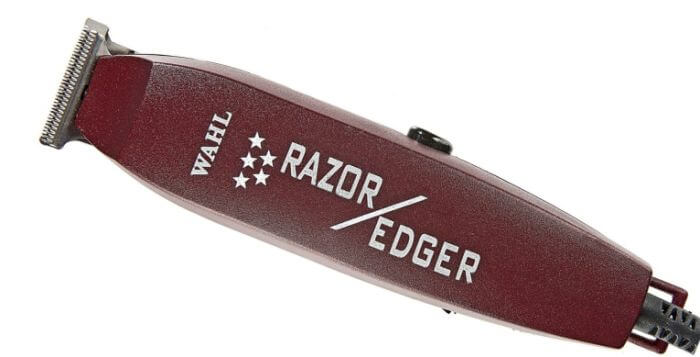The image showcases a vintage-style electric razor and edger by the brand Wahl, W-A-H-L. The trimmer, primarily used for male grooming, is cranberry or maroon in color with a plastic casing. Prominently displayed on a stark white background, the razor is positioned with its metal shaving part in the left corner, angling downward towards the right. The body of the razor features the brand name "WAHL" printed in white, under which five white stars are aligned with three on top and two below. Further down, it reads "razor / edger" in white font. The device has a black switch on the right side and is connected to a black plastic power cord at the bottom. The metal shaving head consists of two sets of teeth that move in a scissor-like action to trim facial hair such as beards, sideburns, mustaches, and stubble.